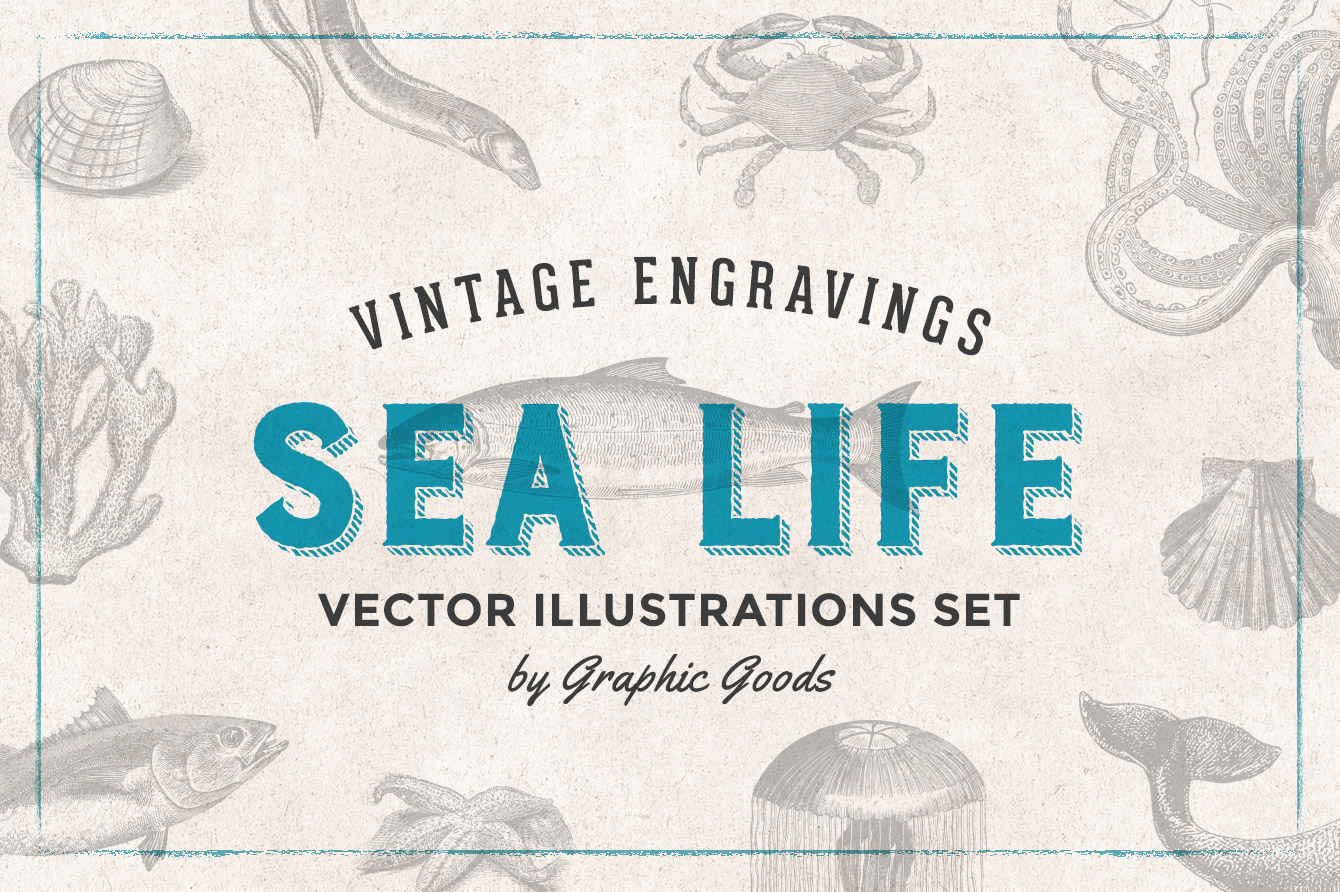This detailed snapshot of a web page is a computer-generated advertisement for a brand called "Vintage Engravings Sea Life." The design mimics the look of vintage paper and features a comprehensive set of gray-toned vector illustrations of various marine animals, including crabs, starfish, fish, octopus, eels, carp, jellyfish, whales, shellfish, oysters, and coral. At the very top, there is a fine blue line border, adding a subtle vintage touch. Dominating the center of the image, "Vintage Engravings" is prominently displayed in capital black letters with a fish illustration beneath it. Overlapping this illustration, the title "Sea Life" is written in a striking turquoise blue, also in uppercase, capturing immediate attention. At the bottom of the image, in black lettering, is the description, "Vector Illustration Set by Graphic Goods." The overall background is gray, enhancing the focus on the intricate sea life drawings and the vibrant title text. The web address is not included in this visual.